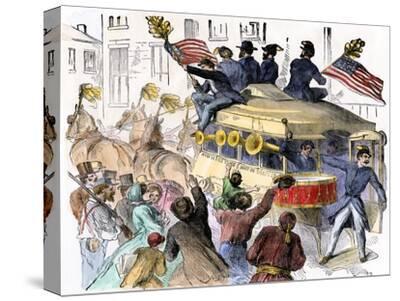The image depicts a vibrant, nostalgic scene, possibly from the Civil War era, animated with the fervor of a patriotic parade. Central to the scene is a grand, horse-drawn chariot progressing forward, pulled by four beige-brown horses. The chariot is bustling with energy as five men sit on top, two of whom proudly wave American flags with golden tops. The men, dressed in blue jackets paired with gray or beige pants, hint at a military presence. A man clad in blue shows partly from a door at the back of the chariot, while another figure peers out from a chariot window.

The chariot itself is festooned with various musical instruments, including trumpets jutting out from windows and a prominent red drum with orange-gold lining. Surrounding the chariot, several women decked out in colorful attire—gray and white, brown, blue-cyan, green, and red dresses—enthusiastically cheer on the parade participants, waving their hats in celebration.

The background subtly reveals the outline of a city, rooting the parade in a historical setting. To the left, armed men and spectators in period costumes suggest a scene from the 1800s, heightening the sense of a bygone era. The detailed illustration captures a lively moment filled with cheering crowds, flag-waving, and the spirited sounds of trumpets and drums.